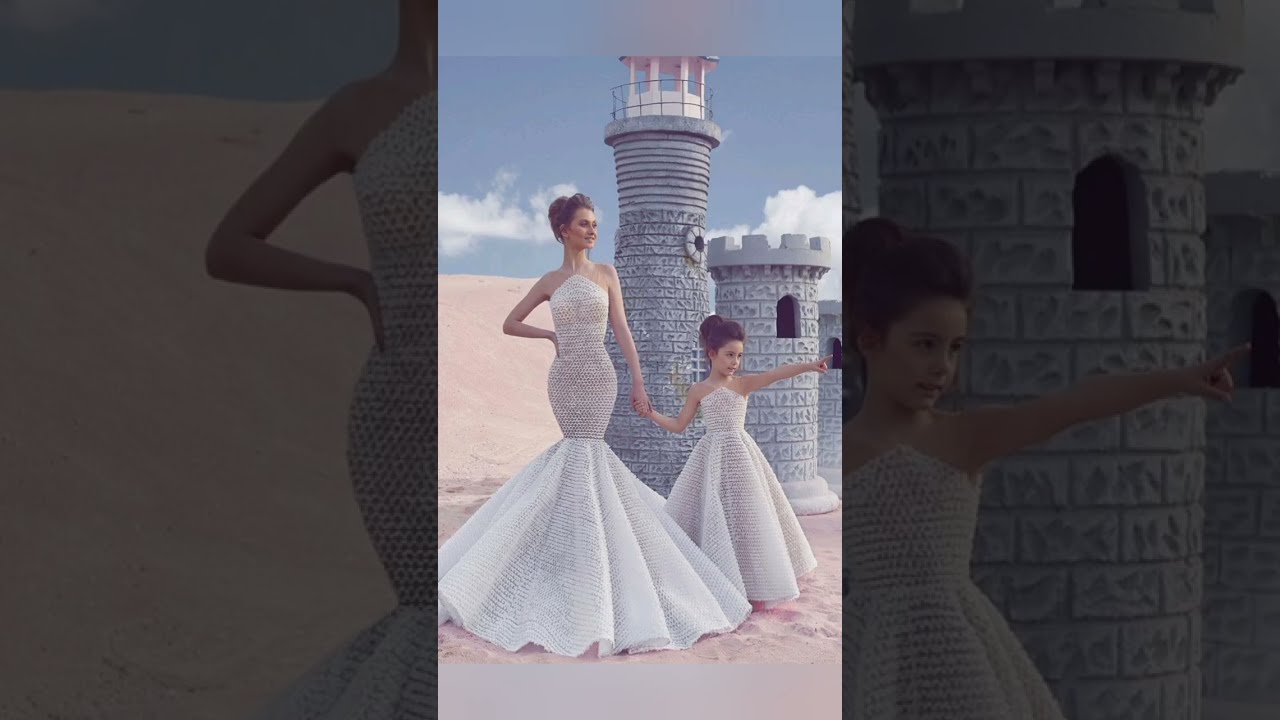In this composite image, three separate photographs merge into one panoramic scene set against a sandy beach with a cloudy, white sky. The central image, brighter and in focus, showcases two prominent structures: a stone lighthouse with a white and red-topped gazebo, surrounded by a wire metal fence, and a smaller, castle-like building with grey stones and arched, open windows.

In the foreground of the central image, an older woman and a young girl are posing in regal, white, form-fitting dresses that flounce out at the bottom. The woman's dress features a mesh top and a mermaid-like, poofy lower half. They stand on the sandy beach, with the girl pointing towards the horizon and the woman smiling, presumably at whatever the girl is indicating. This duo appears touching, akin to a mother and daughter.

Flanking the central image, the left and right photos capture the outer portions of the scene, showing the expanses of the stone structures and the sweeping sandy landscape that includes sand dunes. The structures have a series of round pillars, with the smallest on the right, a medium-sized turret with black, rounded windows, and the tallest forming the lighthouse with its characteristic porthole windows.

Together, these images create a detailed, ethereal scene of familial bonding against a backdrop of historical architectural elements and a beach stretched beneath a vast, cloudy sky.